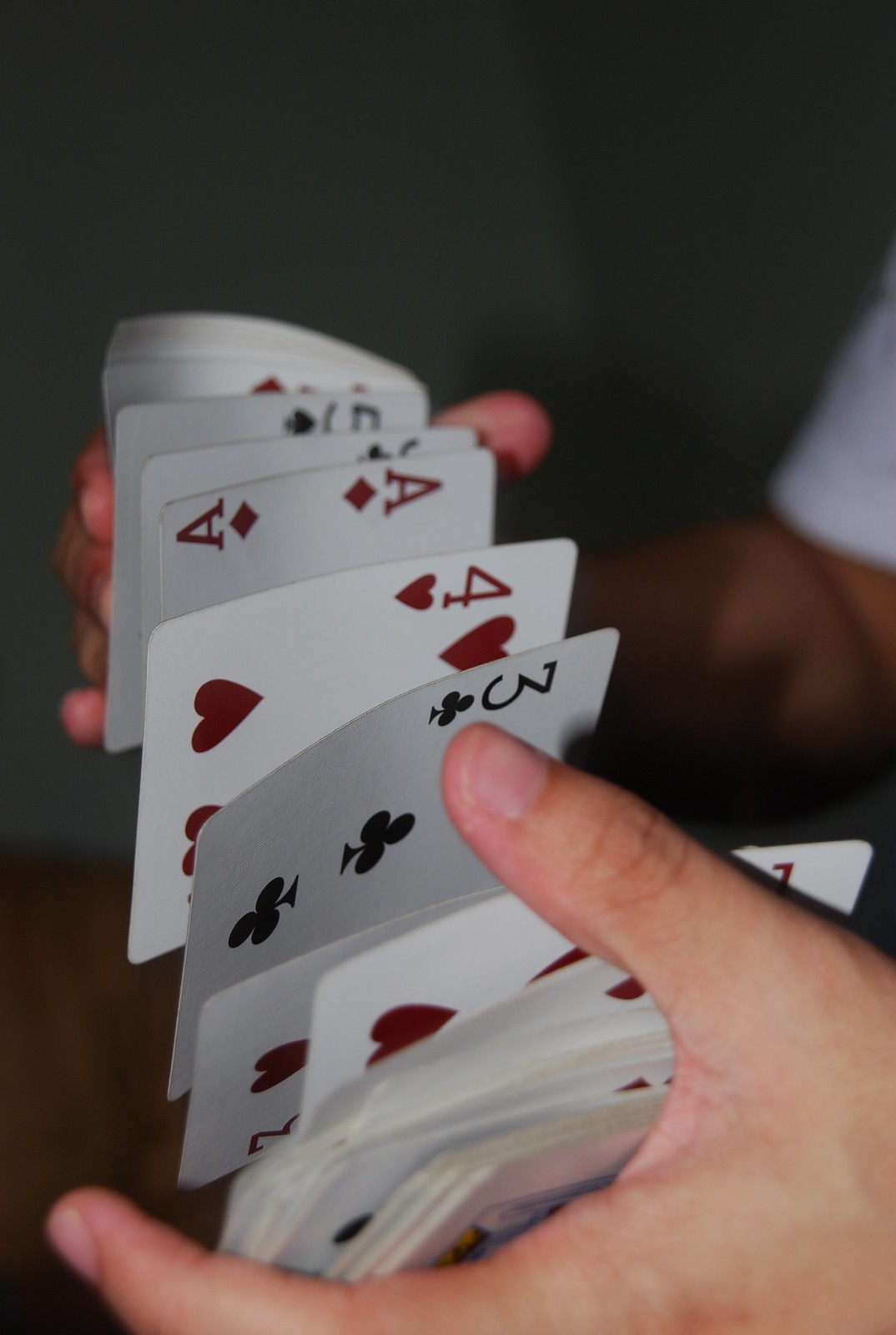In this dimly lit photograph, the skilled hands of a white man are captured mid-action as he expertly shuffles a deck of traditional playing cards. His hands are held apart, with several cards suspended in mid-air, showcasing his professional technique. His right arm, clad in a white short-sleeved t-shirt, is clearly visible, as are the thumb and forefinger of his left hand and the fingers of his right hand gripping the cards. The backdrop is pitch black, adding an air of mystery and focus to the card movement. Detailed among the cards in motion are an ace of diamonds, a four of hearts, a three of clubs, another three of hearts, and a faintly visible five of spades, all set against their white faces, with some cards marked in red and others in black.